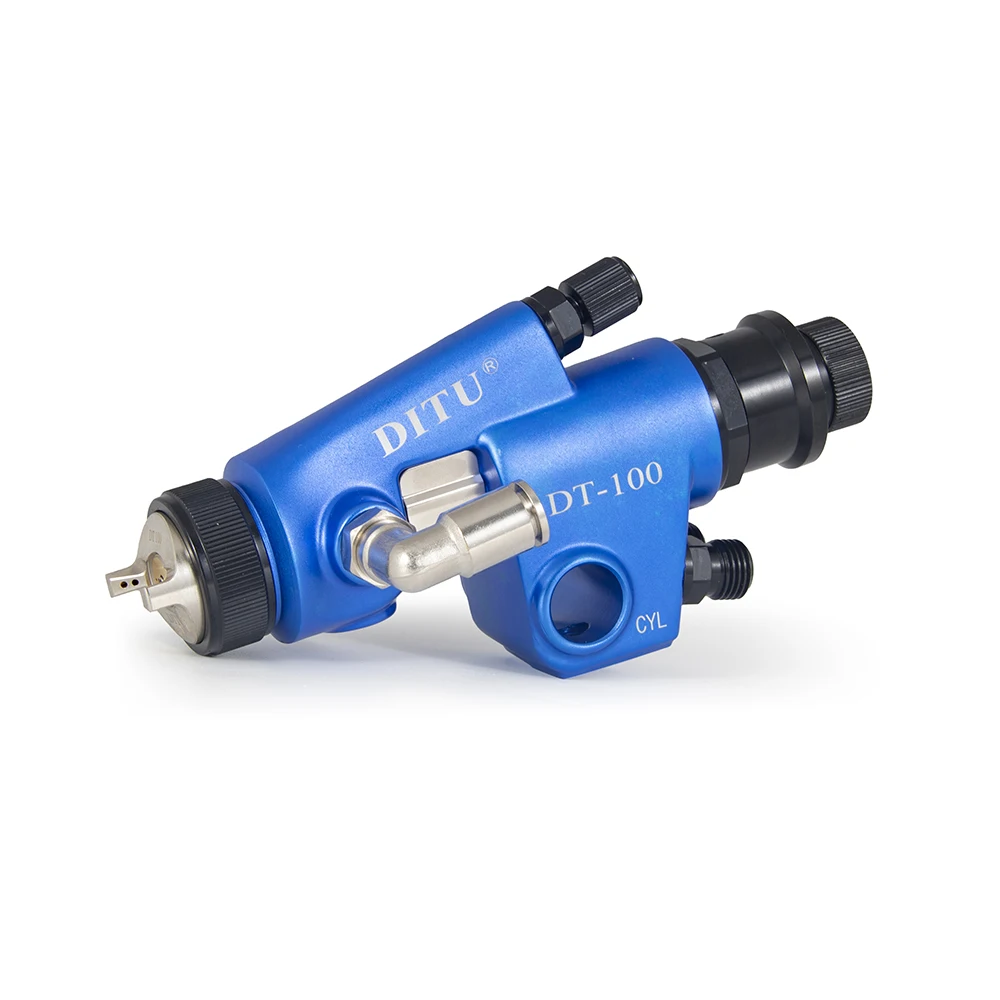This image features a metallic object set against a white background, prominently branded with the term "DITU" and the model designation "DT-100". The object is primarily blue and black with silver elements and bears the inscription "CYL", which likely denotes "cycle". The structure includes various knobs and connectors, some of which are black with ridges to facilitate easy adjustments, and chromatic protrusions. It is oriented towards the left and has an industrial appearance, suggesting it could be a component for machinery, possibly linked to automotive or motorbike mechanics, though its exact purpose remains unclear.